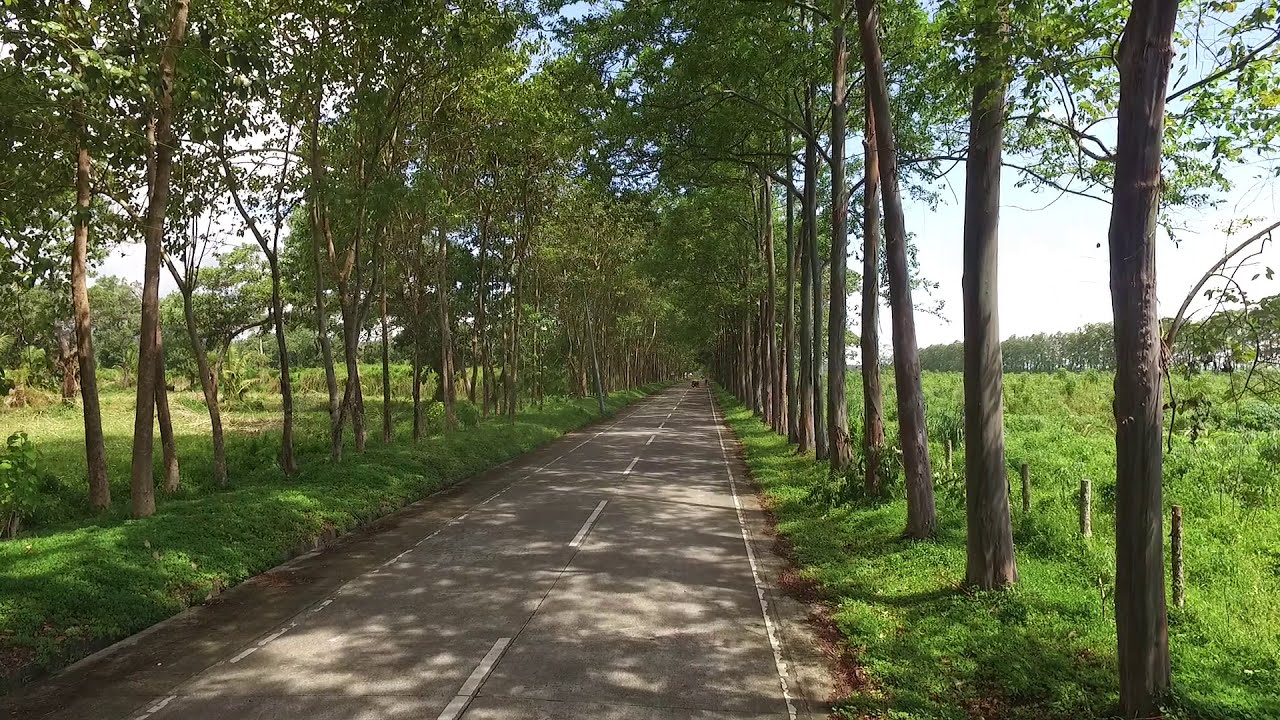The image depicts a serene outdoor setting featuring a two-lane road flanked by tall, leafy green trees that appear to be meticulously planted in neat rows on either side. The road, characterized by its light gray concrete surface, is adorned with white dashed lines down the center and solid white lines along the edges. It stretches into the horizon, gradually converging at a distant point where a vehicle can be observed on the right-hand side. On both sides of the road, well-maintained green grass and shrubs populate the area beneath the trees, contributing to the lush, verdant scenery.

To the right of the road, a field with smaller green plants extends towards a further row of trees, creating a layered landscape of greenery. The left side showcases a similarly green and well-manicured grass area. The ambiance of the image is bright and inviting, with a clear blue sky overhead and sunlight filtering through the tree canopies, casting dappled shadows on the roadway and the surrounding greenery. The interplay of light and shadow creates a picturesque and tranquil atmosphere, emphasizing the natural beauty of the wooded area.